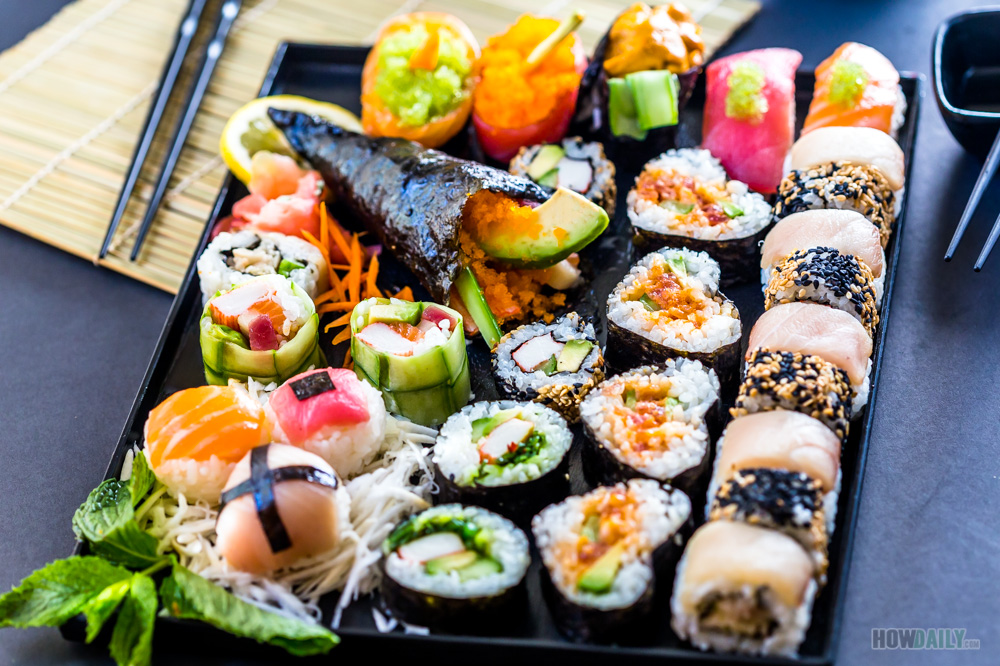The image showcases a meticulously arranged black, square sushi tray, resting on a gray-topped table or a gray tablecloth. The tray is filled with various types of sushi, creating a visually appealing and colorful display. On the right side of the tray, there are five rolls of peach-colored sushi adorned with sesame seeds and topped with salmon. To their left, a set of heart-shaped sushi pieces and further along, some avocado rolls can be seen. The tray also features a conical-shaped sushi with shredded carrots and lemon slice beneath it, topped with orange, couscous-like garnish and avocado slices. In the bottom left corner of the tray, there are three rice balls nestled atop white sprouts with green mint leaves interspersed. The upper right of the image shows a small, square black dish with a pair of black chopsticks resting on it, and another pair of black chopsticks is positioned to the left of the tray on a bamboo placemat. The overall scene is well-lit with natural light, enhancing the vibrant colors and details of the sushi. The image is clear, and in the bottom right corner, the text "howdaily.com" is visible, adding a subtle watermark.